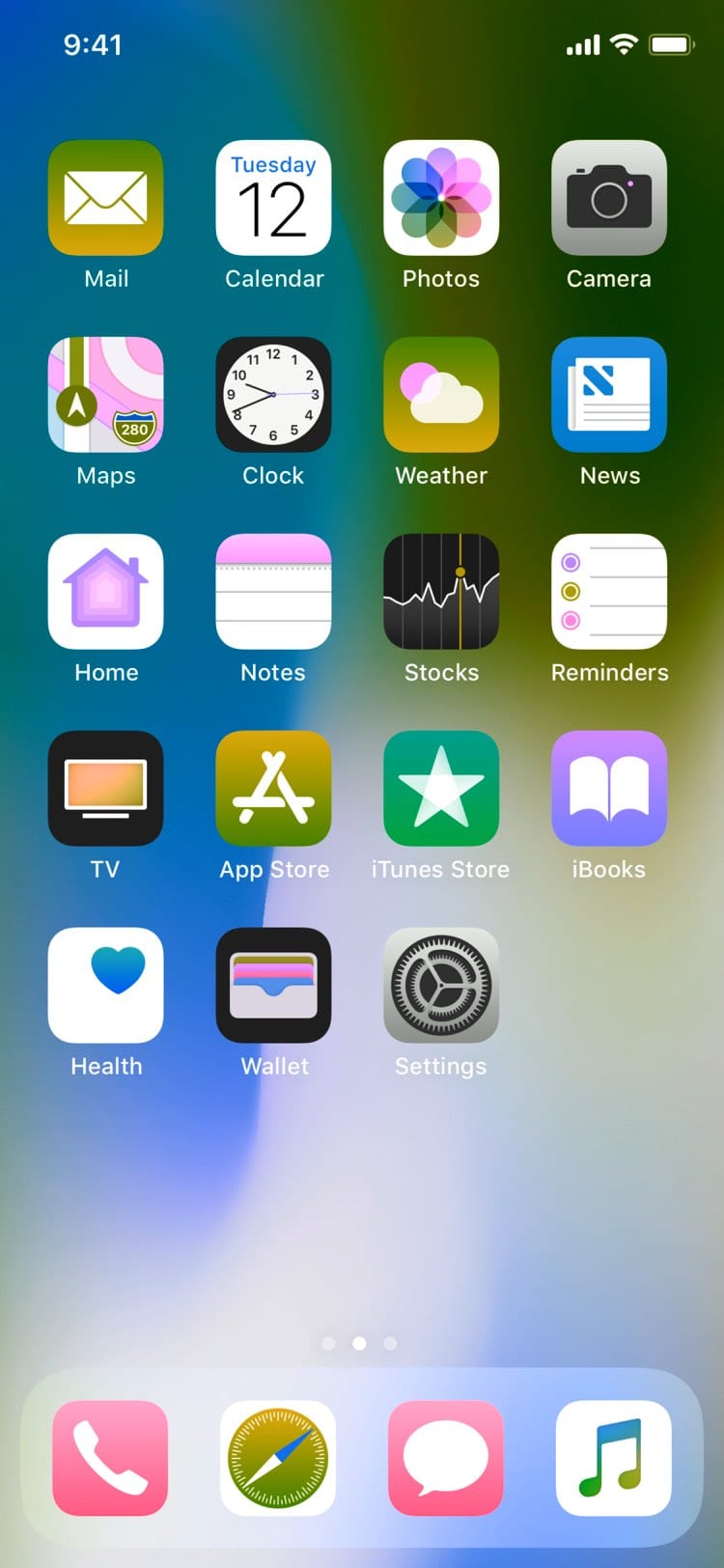This image features a meticulously organized screenshot of an iPhone's home screen, captured at 9:41 AM. At the top of the screen, the status bar displays the time, battery icon, and mobile service indicator. The home screen showcases several rows of app icons, each with distinct, colorful designs that help identify them.

The first row consists of the Mail app, Calendar app, Photos app, and Camera app, positioned from left to right. The second row includes Maps, Clock, Weather, and News apps in the same sequence. In the third row, there are Home, Notes, Stocks, and Reminders apps. The fourth row features the TV app, App Store, iTunes Store, and iBooks.

Further down, the fifth row displays the Health app, Wallet app, and Settings app, which are essential for various functionalities. Notably, four frequently used apps are strategically placed in the dock at the bottom of the screen for easy access. These apps include the Phone app, which is likely Safari due to its compass-like design, the Messages app, and the Music app.

Overall, the apps are neatly arranged, presenting a well-organized digital workspace on the iPhone.